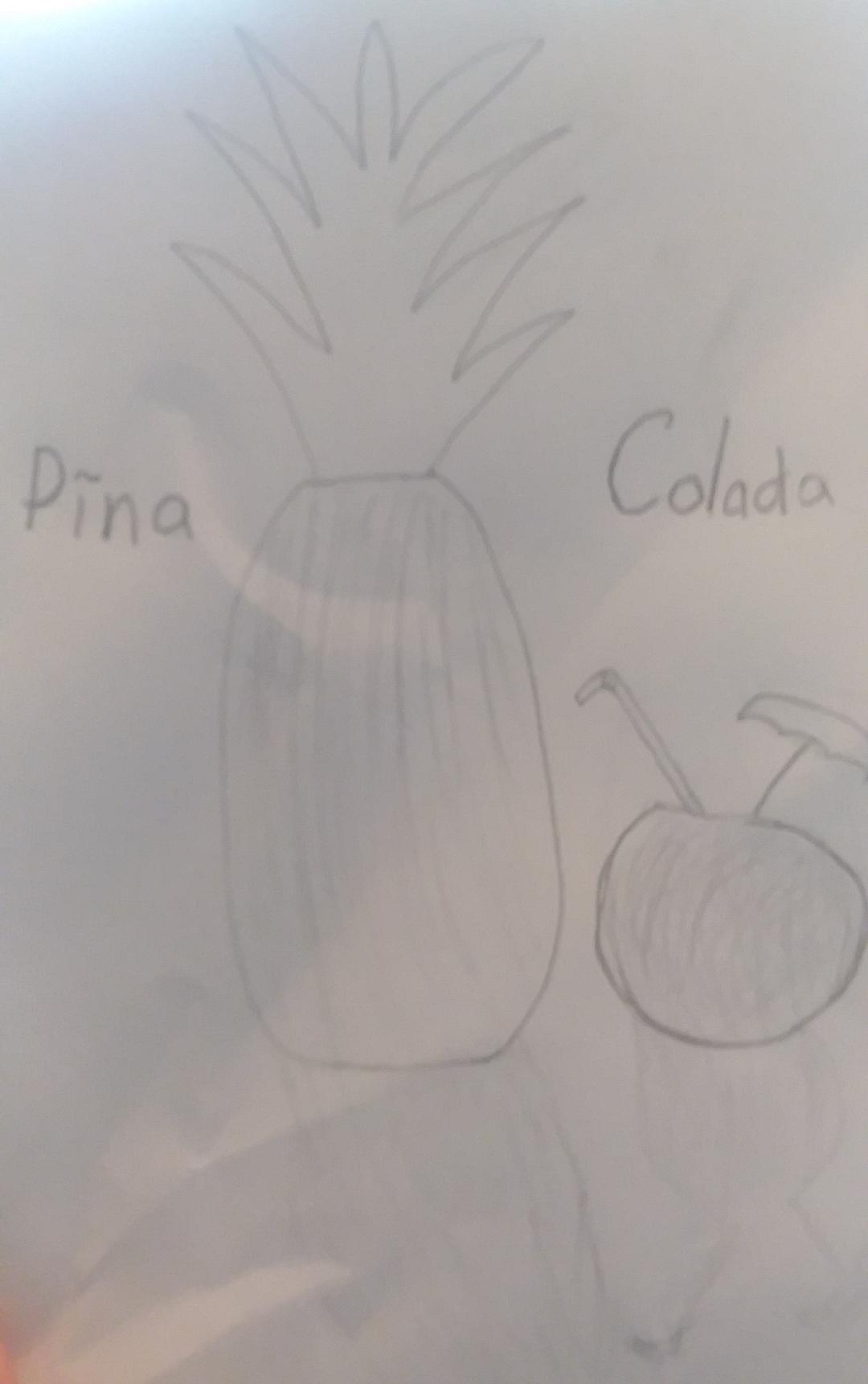This detailed sketch features the word "PINA" on the left, followed by the word "COLADA" on the right, both rendered in a soft gray hue. Between these words lies an intricate drawing of a pineapple. The pineapple begins with a vertical, oval shape and transitions into a series of zigzag lines at the top, capturing the texture and spiky leaves typically seen on a real pineapple. Below the "PINA COLADA" text, there is a circular object resembling a cocktail, complete with a straw protruding from the left side and a miniature umbrella from the right, suggesting a refreshing tropical drink. The entire illustration is outlined in gray, set against a gray background that features a subtle hint of light blue light illuminating the top left corner, adding a gentle touch of color to the composition.